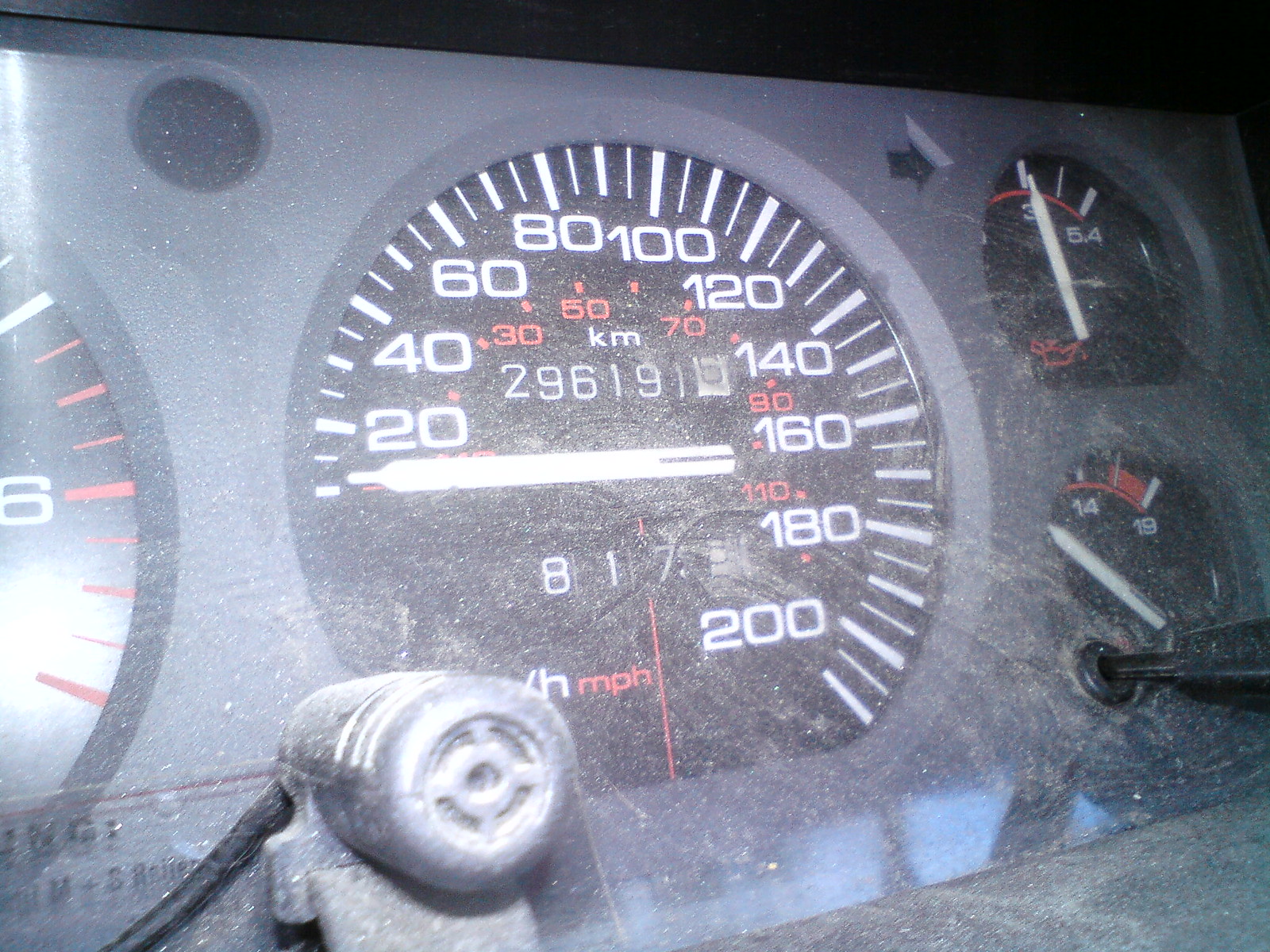This nighttime photograph captures the detailed dashboard of a vehicle, with emphasis on the speedometer, which prominently displays both kilometers per hour and miles per hour. The primary scale is in kilometers per hour, ranging from 0 to 200. The odometer indicates that the vehicle has accumulated 296,196 kilometers, suggesting it has seen extensive use. Additionally, the trip meter reads 817 kilometers.

On the lower right of the dashboard, a voltage gauge is visible, while the upper right features an oil pressure gauge. To the left edge of the image, a partially visible tachometer hints at the full dashboard layout, though it is cropped out in this landscape-oriented photo. The dark background and the illumination provided by the camera suggest the picture was taken at night. The speedometer needle resting at zero confirms the vehicle is stationary.